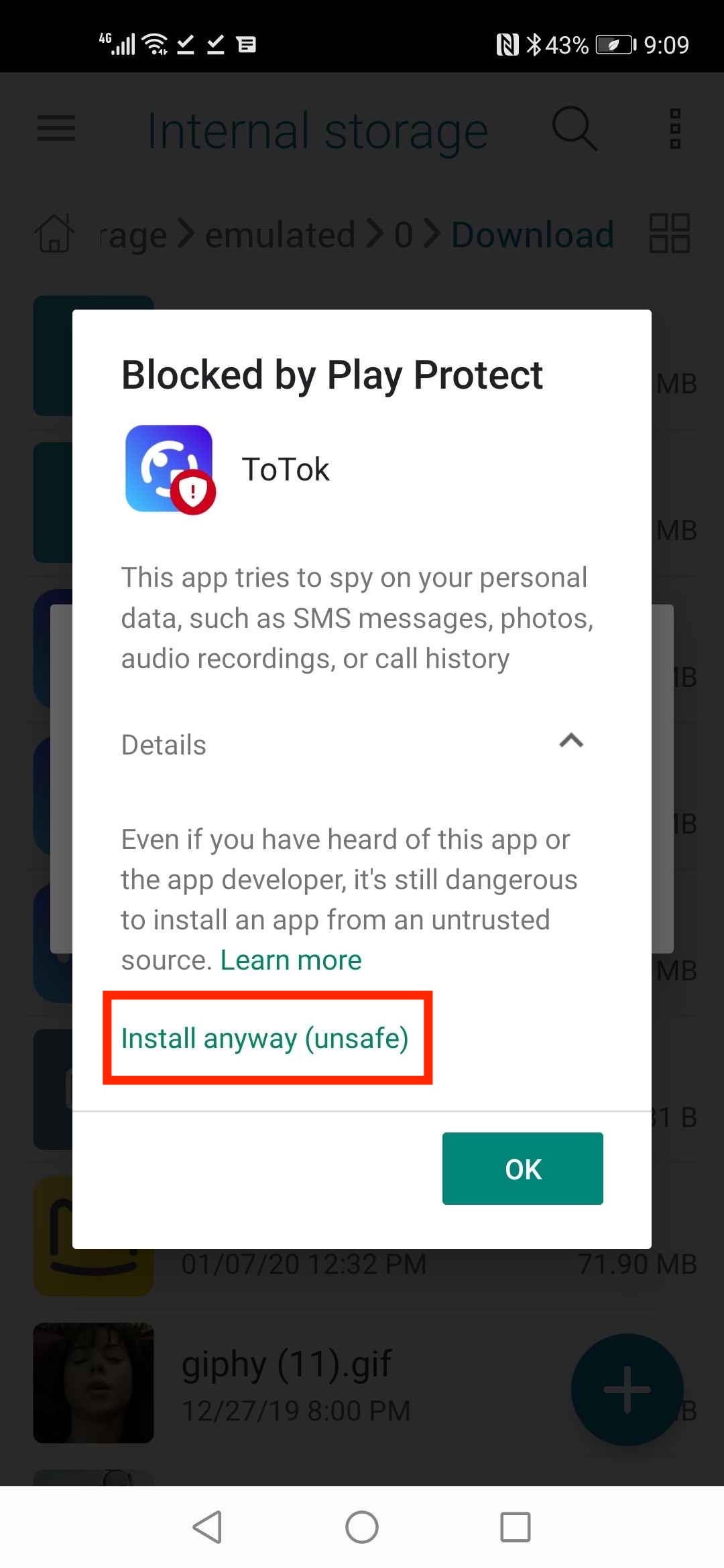The image portrays a notification on an Android device issued by Google Play Protect, warning the user about an unsafe app named "Totalk." The warning advises that the app has been blocked due to its potential to spy on personal data such as SMS messages, photos, audio recordings, and call history. 

The notification includes a detailed drop-down option, and a message urging caution even if the user is familiar with the app or its developer, emphasizing that it's dangerous to install apps from untrusted sources. A green hyperlink labeled "Learn more" is provided for additional information.

Below this, the notification presents an "Install anyway" button marked as "unsafe" in parentheses, which is highlighted in red. Additionally, there is a green "OK" button at the bottom of the dialog box. 

The overall layout of the warning dialog box, featuring various icons and text elements, is centered on the screen. The inclusion of the "Install anyway" button suggests that the creator of the screenshot might be demonstrating how to bypass the Play Store's security warnings, despite the associated risks. The image serves as a cautionary note about bypassing security measures to install potentially harmful applications.